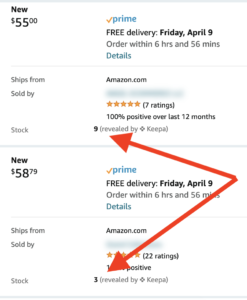In the image, there are two product listings being compared side by side. 

The first listing, located at the top, features a new item priced at $55 with Prime Free Delivery expected by Friday, April 9th. Customers are encouraged to place their orders within 6 hours and 56 minutes to qualify for the delivery date. The item ships from Amazon, but the seller's name is blurred out. It boasts a perfect 5-star rating based on 7 reviews, with a 100% positive rating over the past 12 months. A red arrow points to "Stock 9," information revealed by Keepa.

The second listing, displayed below the first, shows a new item priced at $58.79, also with Prime Free Delivery available by Friday, April 9th, and the same ordering time frame of 6 hours and 56 minutes. This item also ships from Amazon and has the seller's name blurred out. Similarly, it has a 5-star rating but from a larger pool of 22 reviews. The positive rating percentage is obscured by another red arrow, but it appears to indicate 100%. This arrow directs attention to "Stock 3," information also revealed by Keepa.